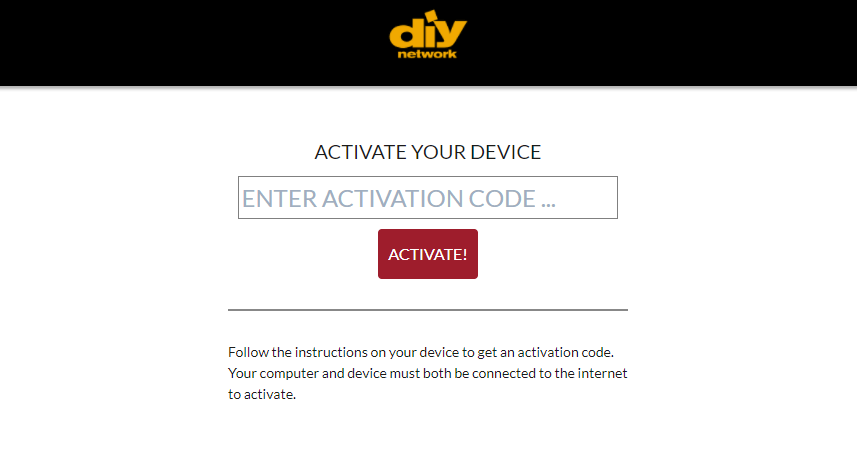The image displays an activation code screen for the DIY Network. At the top of the screen, "DIY Network" is prominently featured in bold orange text set against a black rectangular background. Below this, the rest of the image has a clean, white background. 

Headlining the content, the phrase "Activate Your Device" is written in clear, black text. Directly beneath this header, there is a designated gray-text rectangle with the placeholder text "Enter activation code...". This is where users are prompted to input their activation code. Following this section, a bright red square button centrally positioned contains the word "Activate" in bold, white text inviting the user to proceed with the activation process.

A thin black line is placed under the red button, delineating the main interactive elements from the informational text below. At the bottom of the image, there are further instructions: "Follow the instructions on your device to get an activation code. Your computer and device must both be connected to the internet to activate," written in black text, ensuring users understand the necessary steps and conditions.

The entire screen is laid out on a white background, providing a clean and straightforward user interface. This description captures the completeness of the activation screen from top to bottom.